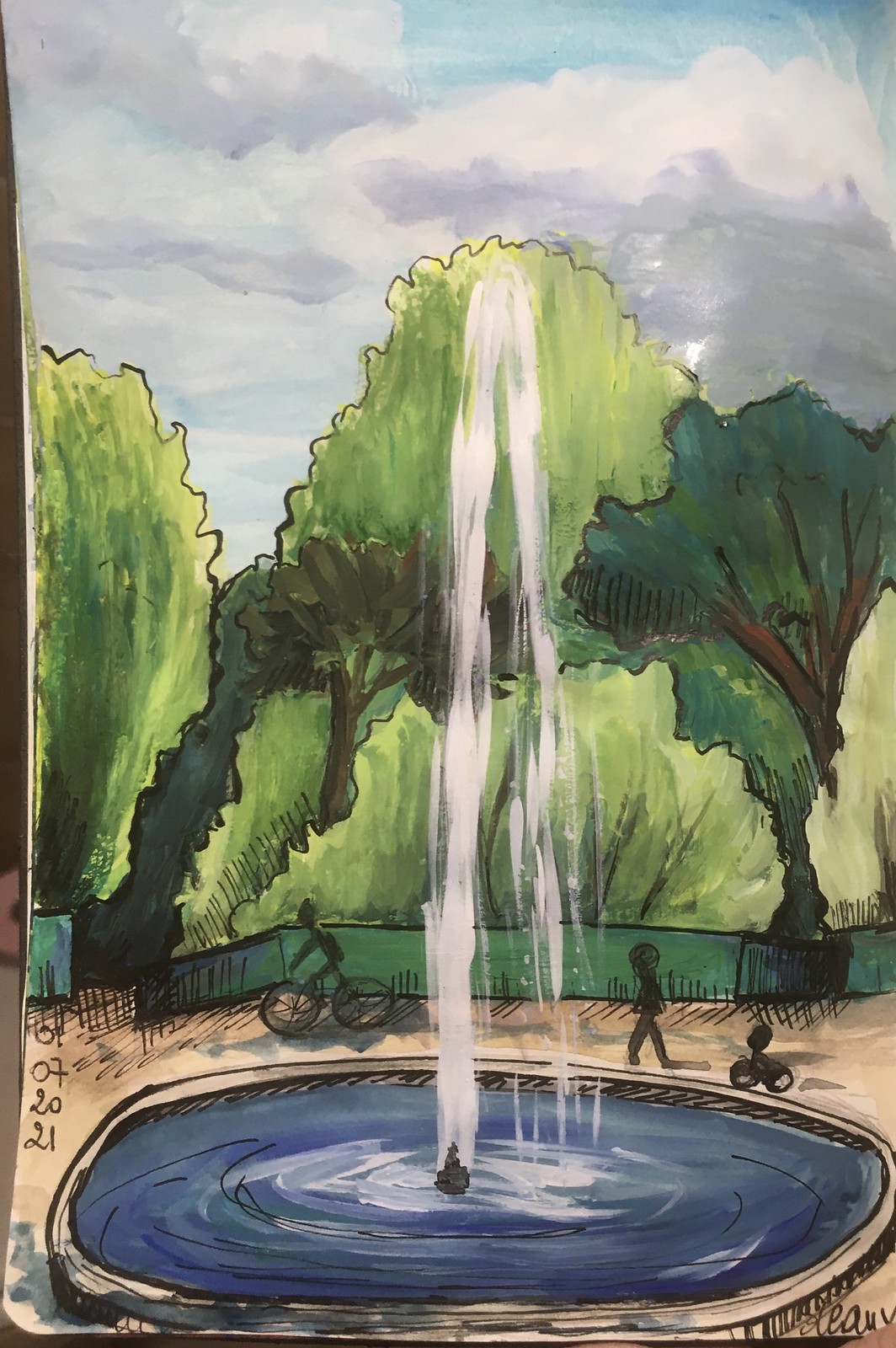A surreal painting depicts a whimsical fountain at its center, dominating the composition. The fountain, with a bluish base, intricately designed yet rendered in an abstract manner, releases a pristine white spray of water. The water arcs gracefully towards the sky before cascading back down. At the rear side of the fountain, within the watery basin, two stick figure-like characters add an intriguing element to the scene. One figure rides a bicycle while the other, possibly a child, follows closely behind on what appears to be a tricycle. The background features an imaginative landscape with varying hues of green, suggestive of grass or tree formations. Overhead, the sky is filled with brooding, gray clouds, lending a fantastical yet tranquil atmosphere to the entire painting.